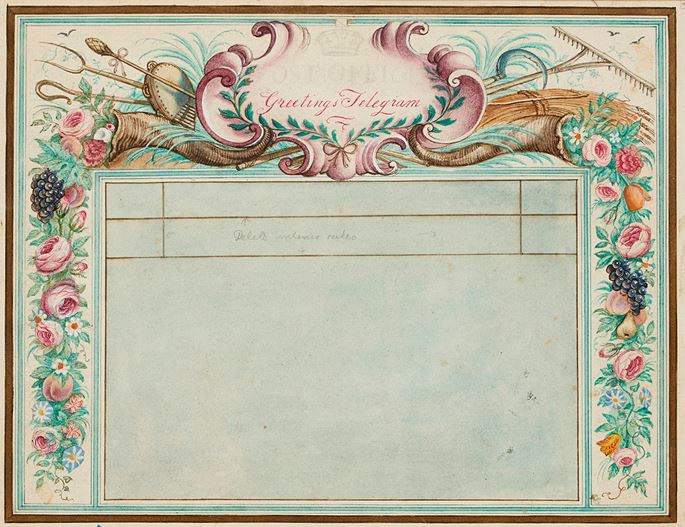This image depicts an old-fashioned telegram style announcement, likely from the early 20th century, featuring a prominently detailed and ornate design. The document is rectangular and portrays a sense of antiquity with a slightly dirty and faded appearance. It is framed by a gold border at the very edge. The central focus at the top of the image is the phrase "Greetings Telegram" in a distinctive pink script font. 

Below this title, the page is adorned with an intricate floral and musical motif. On each side of the telegram, there are elaborate designs that include a variety of flowers in shades of pink, orange, and blue, as well as bunches of purple grapes. Interwoven among these elements are images of musical instruments such as a bugle, and decorative items resembling a cornucopia from which the flowers spill out, alongside shell-like designs in pink that accentuate the curls and vines of the composition.

The actual space designated for the telegram message takes up approximately 70% of the page and is centered towards the bottom. This area, tinted in a faded blue, suggests where the personal message would be written, though it appears somewhat obscured due to the age-related wear and tear of the document. The thorough detailing around this space highlights the significance and celebratory nature of the telegram, enhanced further by the overall pastel-colored and ornamental design.